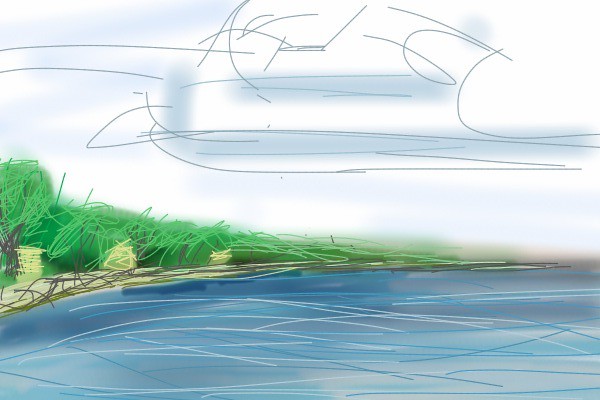The image depicted is a highly artistic and abstract color composition, reminiscent of a painting. At the top, a white sky is subtly streaked with shades of grey, creating a moody and textured backdrop. Grey horizontal columns and diffuse grey patches dominate the left side, layered with black penciled lines that form an indecipherable, chaotic pattern. In the left middle section, abstract foliage or tree-like shapes emerge, characterized by their narrow and thin leaves. These trees appear to border a coastal area, perhaps along a river or lake. Below them, smaller, lighter shrubs can be seen. The ground features a kind of pavement area with greyish scribbles, adding to the abstract landscape. At the bottom of the image, a body of water in shades of blue and grey is visible, further enhanced by light grey and blue scribbled lines, creating an overall diffuse and dreamy aesthetic.